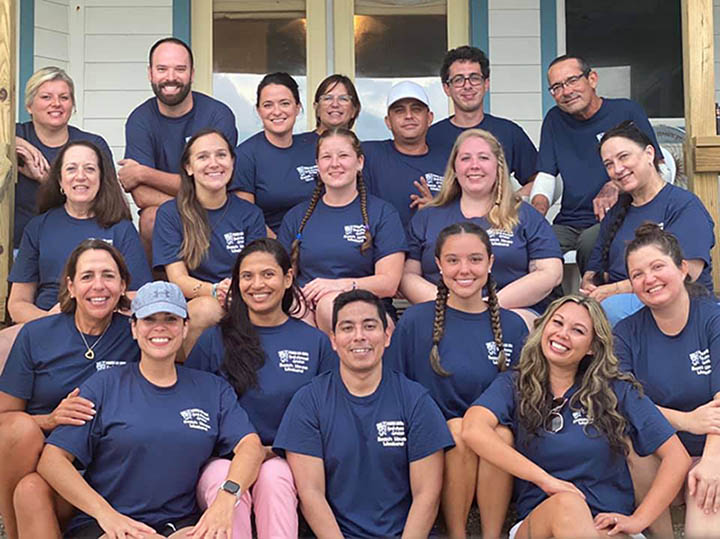The image captures a large group of mostly young men and women, likely in their twenties, gathered in front of a building with white siding, blue trim, and pale yellow doors. They are sitting on steps, arranged in a staggered formation, suggesting multiple rows. The group appears to be part of an organization or volunteer club, as they are all wearing matching royal blue t-shirts featuring a white logo or paragraph of text over the left side of the chest. Some individuals in the group are wearing hats, including ball caps, and there is a mix of long and short hairstyles, predominantly dark brown and black hair. The building behind them has a porch supported by light brown wood posts and includes a set of yellow doors with glass windows, enhancing the communal and friendly atmosphere of the scene.